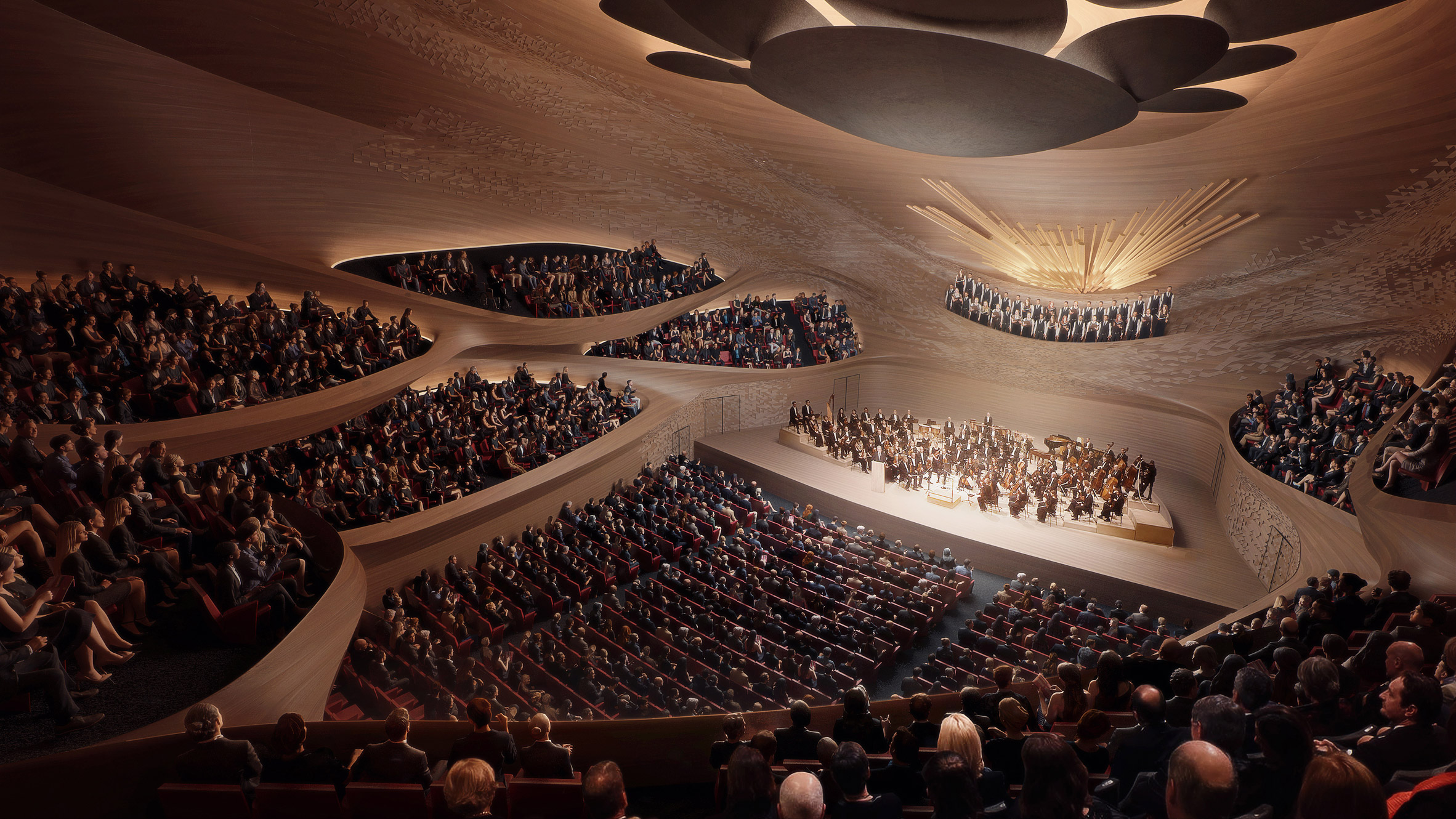This image captures an overhead view of a modern, expansive performance hall taken from the highest balcony tier. The concert hall is filled to capacity, with every seat occupied by spectators. The hall is characterized by its undulating light brown ceiling adorned with large gray ovals and a central light fixture emitting light from behind. The audience seating features sections on the main floor, a first balcony, and a second balcony. The seats are arranged in long rows, with the floor seats being darker in color, possibly dark red or brown, and the overall layout forms circular and oval groupings around the hall.

On the stage, which is tan and surrounded by curved wooden railings, sits a symphony orchestra, all dressed in black and illuminated by golden lighting. Although the musicians are distant and indistinguishable from one another, their presence is dominant on the main floor section of the stage. Behind the orchestra, there are two elevated tiers where a choir of roughly 30 to 40 people, also dressed in black, stands. They are positioned in front of an art installation resembling sunrays made from golden sticks. The entire scene is a harmonious blend of modern architectural design and classical music performance, unified by the dynamic, flowing lines of the ceilings and the strategic placement of lighting.